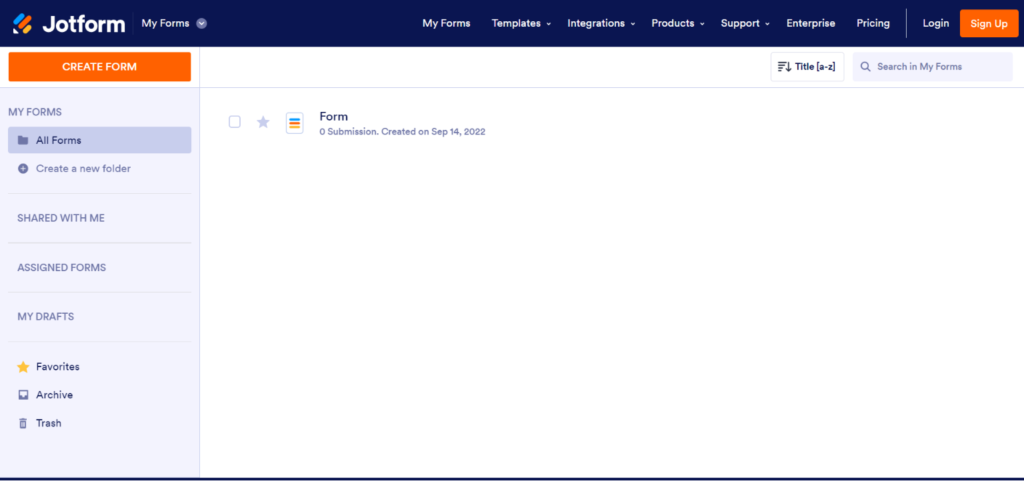The image appears to be a screenshot of a JotForm dashboard page. The top part of the screen has a gradient background transitioning from navy blue to purplish blue. In the upper left-hand corner, the text "JotForm" is written in white with a capital "J," followed by "MyForms" directly beneath it. 

Directly to the right of "JotForm MyForms," there is a menu bar with white text options: "My Forms," "Templates," "Integrations," "Products," "Support," "Enterprise," "Pricing," and "Login." To the far right, there's an orange rectangular button with "Sign Up" written in white text.

On the left side of the page, beneath the header, there is another orange rectangle with the white text "Create Form." Below this, in light purple text, it says "MyForms," followed by a list of navigation options: "All Forms" (highlighted in darker purple), "Create a New Folder," "Shared With Me," "Assigned Forms," "My Drafts," "Favorites," and "Archived Drafts."

On the right side, there is a white rectangular box at the top. In this box, in black text, it reads "Title A to Z." Beneath it, there is a light purple rectangular search bar with a light purple magnifying glass icon and the text "Search in MyForms."

Below the search bar, along the left side, there is a white box outlined in light purple. Inside this box, there are multiple lines in different colors: a blue line, a red line, and a yellow line. Next to this, in black text, it says "Form." Below this, there is text that reads "Zero Submission Period Created on SEP 14," indicating the creation date of September 14th, 2022.